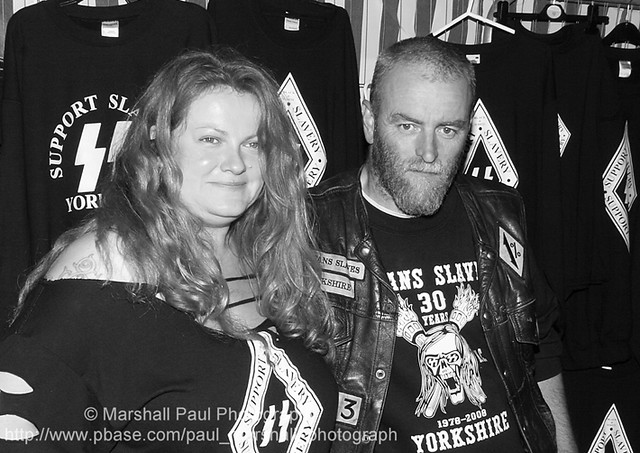In this black and white photograph, two individuals are seen standing indoors, posing for the camera. The woman on the left, with long hair, is slightly smiling and wearing a black t-shirt that features a design. The man on the right, with a shaved head and significant facial hair, wears a black t-shirt with a skeleton head design and some text, along with a biker jacket adorned with various symbols. The text on his shirt reads "1978 to 2008" and "Yorkshire," while other prominent features on their attire include white supremacist symbols such as SS symbols and a "one percenter" diamond. In the background, several t-shirts hang from hangers. At the bottom left of the image, there is a watermark that reads "Copyright Marshall Poll www.pbase.com," with additional text partially obscured due to low color contrast.